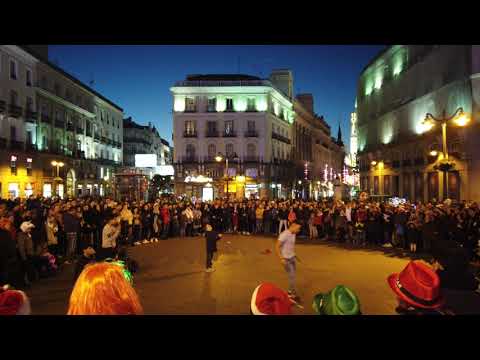In the heart of a bustling city square, framed by tall, white buildings adorned with numerous windows and balconies, a vibrant scene unfolds under the night sky. The deep blue of the dusk contrasts with the glowing yellow and white streetlights, casting a colorful illumination over the area. An open space at the center of the square is filled with energy as two men in white T-shirts and blue jeans engage in an animated dance, possibly a dance battle or street performance. This lively display has attracted a crowd, with spectators wearing distinct green and red hats and one with striking orange hair, gathered closely around the performers. The atmosphere feels international, perhaps reminiscent of a town square in France or London, where the buildings, reaching up to five stories high, surround the lively spectacle at street level.